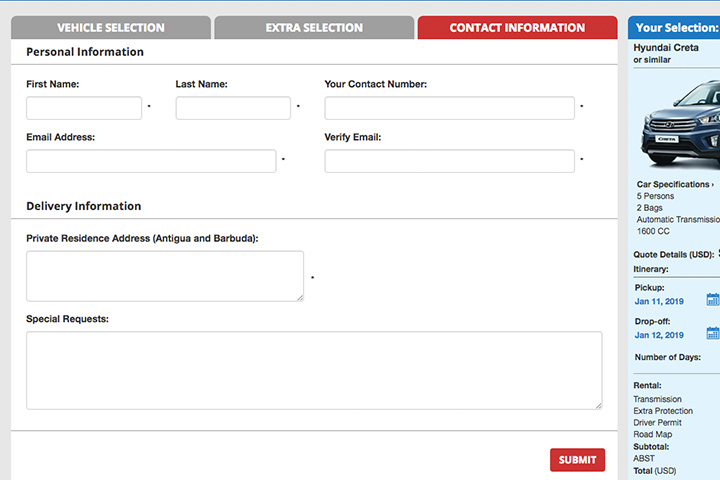The image is a screen capture of a car rental website. At the forefront is the "Contact Information" tab, which is currently selected. Two other tabs, "Extra Selection" and "Vehicle Selection," are also visible.

In the "Contact Information" tab, the following fields are listed under "Personal Information": First Name, Last Name, Contact Number, Email Address, and Verify Your Email, all of which are marked as required fields. 

Furthermore, there is a section for "Delivery Information," asking for a private residence address. However, the text appears jumbled, making it unclear whether the address should be in Antigua and Barbuda or some other place.

Additionally, there is a space designated for "Special Requests." On the right side of the screen, there is a summarized section titled "Your Selection," indicating that a Hyundai Crèssta, or a similar vehicle, has been chosen.